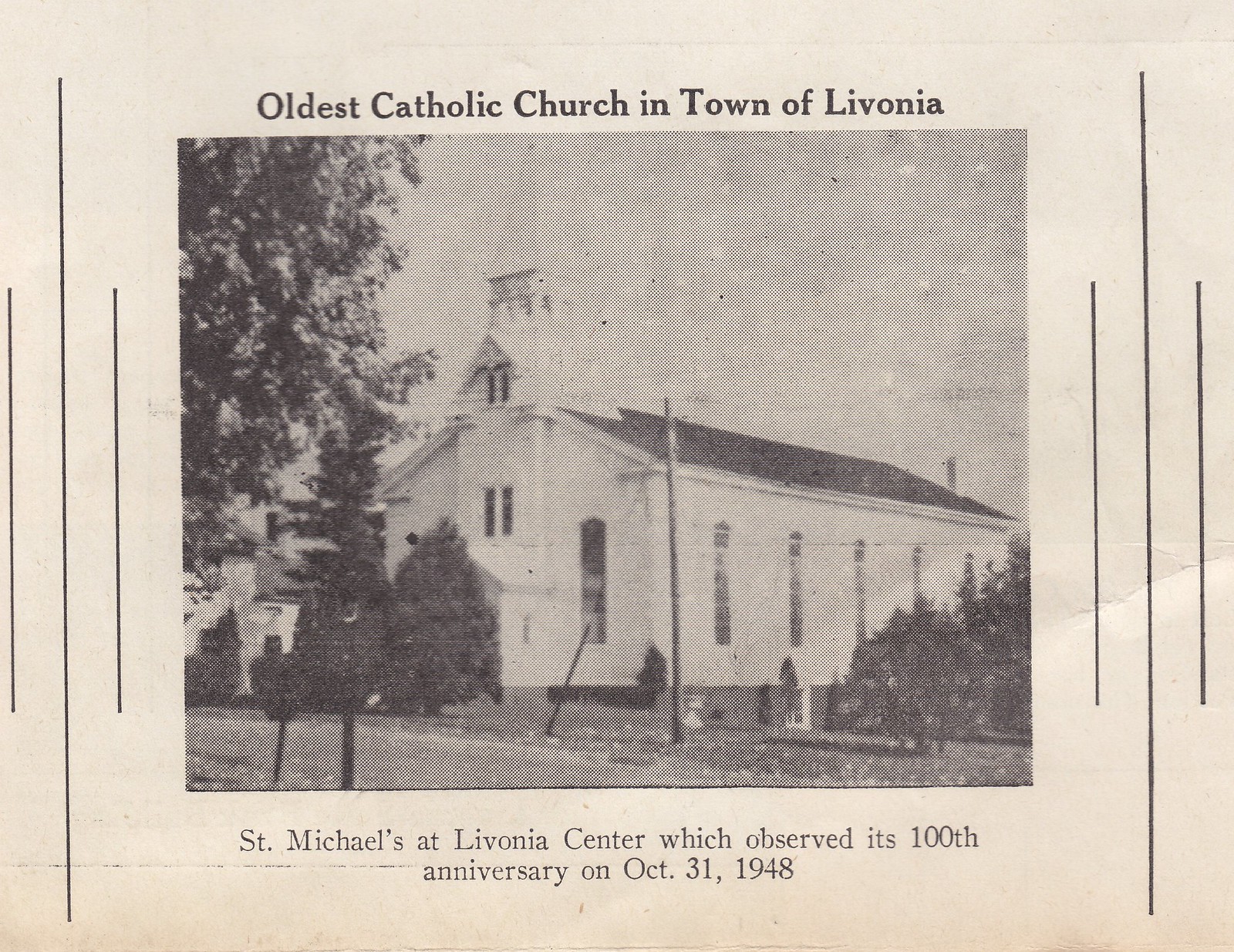This image features a rectangular-shaped, black-and-white photograph centrally positioned against a cream-colored background. The photograph appears to be very old, potentially from the 1940s, and resembles something that might have come from a newspaper or old publication. The picture showcases the exterior of St. Michael's at Livonia Centre, recognized as the oldest Catholic Church in the town of Livonia. Inscribed at the top of the photograph is the text, "Oldest Catholic Church in Town of Livonia," while at the bottom it reads, "St. Michael's at Livonia Centre, which observed its 100th anniversary on October 31, 1948."

In the photograph, the white church building stands amidst trees, with a large chimney and the steeple positioned on the left side of the structure. Adjacent to the church is a telephone pole, and the surrounding area is covered with grass. The image colors are predominantly white, gray, and black, enhancing its vintage feel. Adding to the historical ambiance, three vertical black lines are present on both the left and right sides of the image.